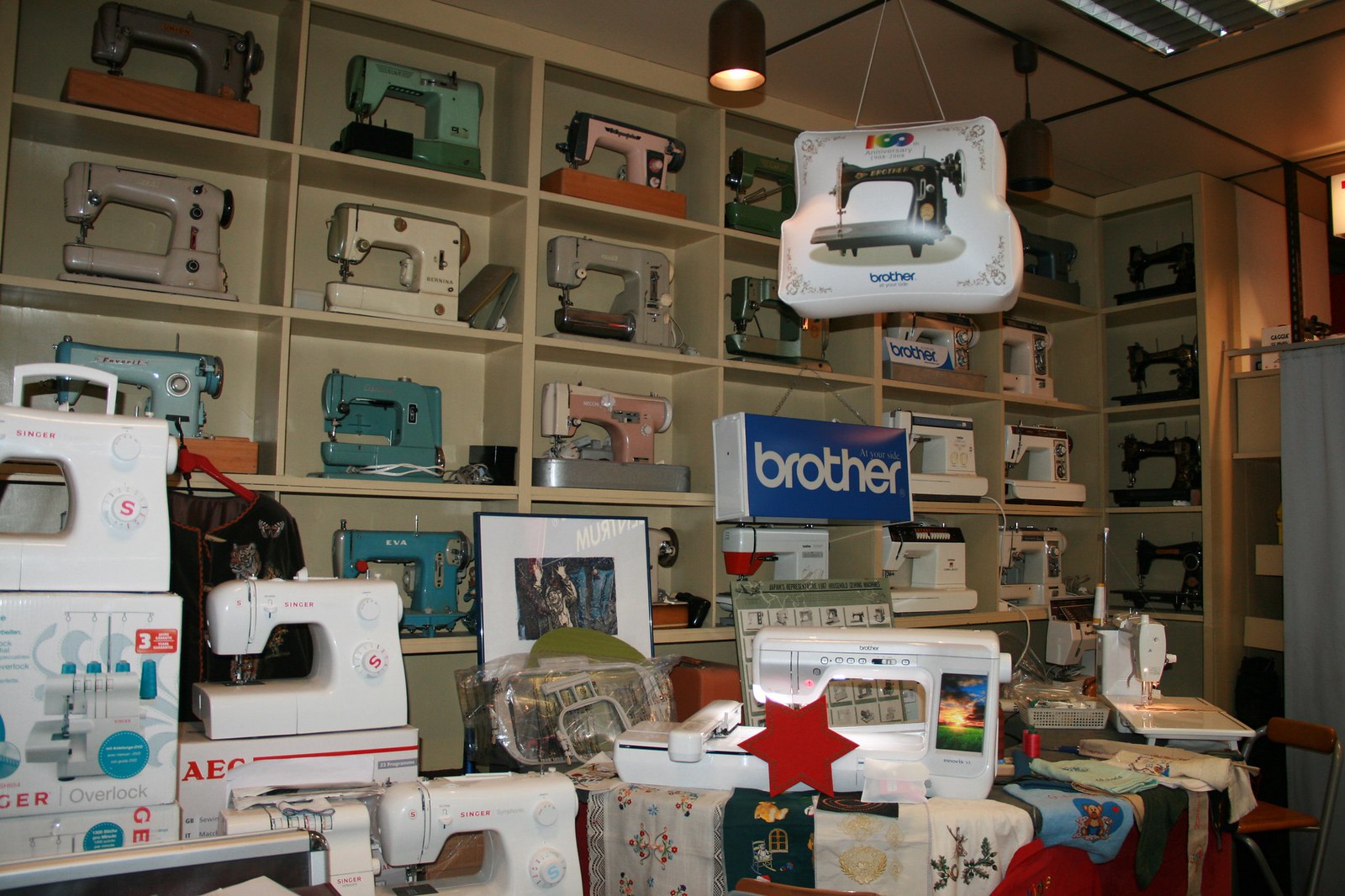The image depicts an indoor scene with a somewhat dark, amateur photo quality. It appears to be taken in a space that could be a store, museum, or factory, primarily featuring a collection of Brother sewing machines. The wall is lined with built-in shelves, each bearing an individual sewing machine in various colors including pink, blue, turquoise, tan, green, gray, and black. Prominently, there are two light fixtures—one illuminated and one off—enhancing the room's varied lighting. A balloon displaying a sewing machine with the text "100" above it and "Brother" in blue beneath can be seen, reinforcing the brand's prominence. Centered in the room is a blue sign reading "Brother," suggesting the emphasis on Brother sewing machines. Alongside the wall of shelves, multiple tables are adorned with multicolored tablecloths in blue, white, and red hues, further stacked with additional sewing machines and several boxes. The assortment includes a range of vintage to modern models, with the vintage machines notably displayed on the far right shelves.